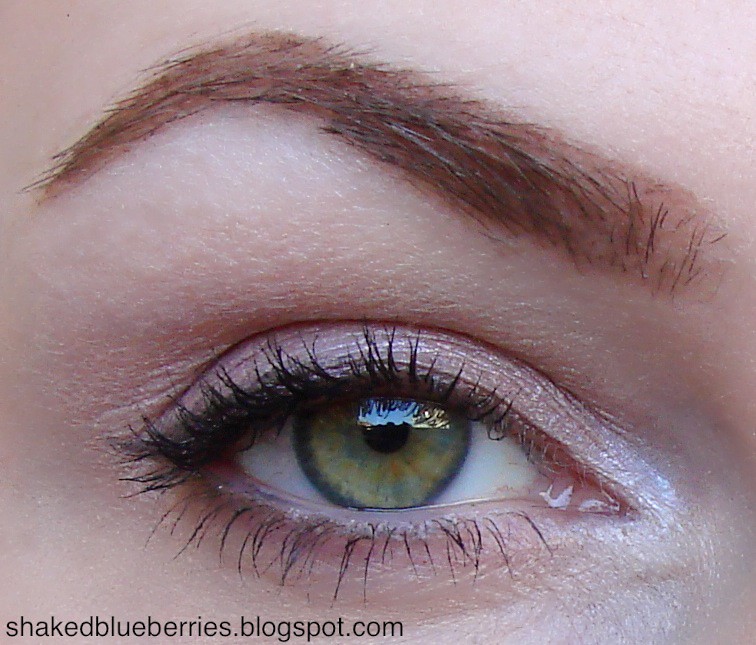The close-up image features the right eye of a white woman, highlighting detailed features such as a well-trimmed, arched eyebrow with brown hairs. The eye is framed by neat, possibly mascara-coated eyelashes, and the pupil within the open eye appears brown, contrasted by hazel green tones in the iris. The focus of the image is intensely directed straight ahead, giving a sharp and attentive look. At the bottom of the image, the text "shakedblueberries.blogspot.com" is visible, serving as a watermark in black text. This striking and detailed close-up emphasizes the natural and meticulously groomed aspects of the eye.